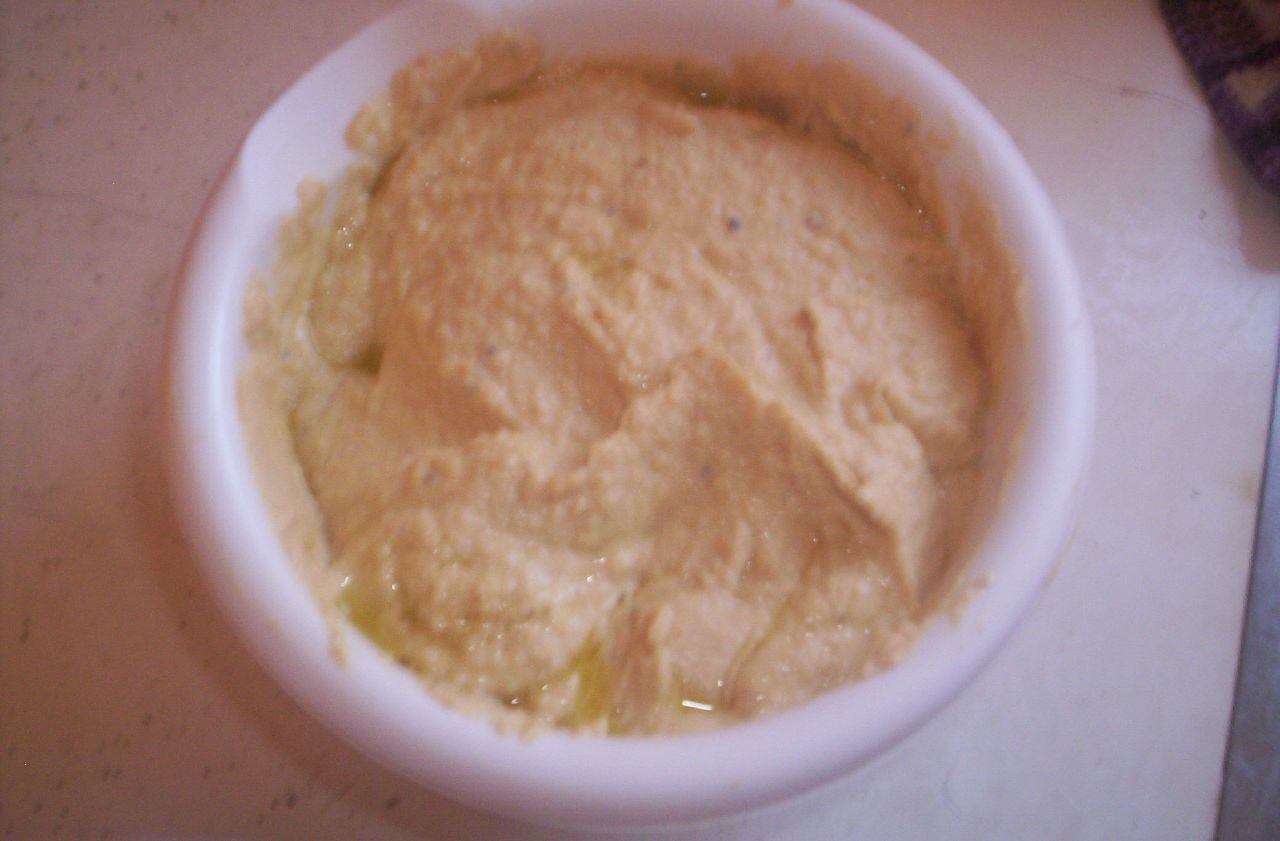The image centers on a small white bowl positioned on a white surface that appears to be a table. The main content of the bowl is a yellowish mixture, resembling hummus or perhaps a kind of porridge, with hues of light orange, tan, and some slightly yellow spots. Lying beneath the bowl, the surface has a sheen, suggesting possible traces of oil. The backdrop on the left side is pink, darkening towards the bottom, while the right side transitions from pink at the top to white with a brown patch in the upper right corner and a small spill of lighter brown below it. Additionally, the bottom right corner of the image features a tall gray triangle. Overall, the photograph is rectangular and likely taken in an indoor setting, capturing the close-up details vividly.